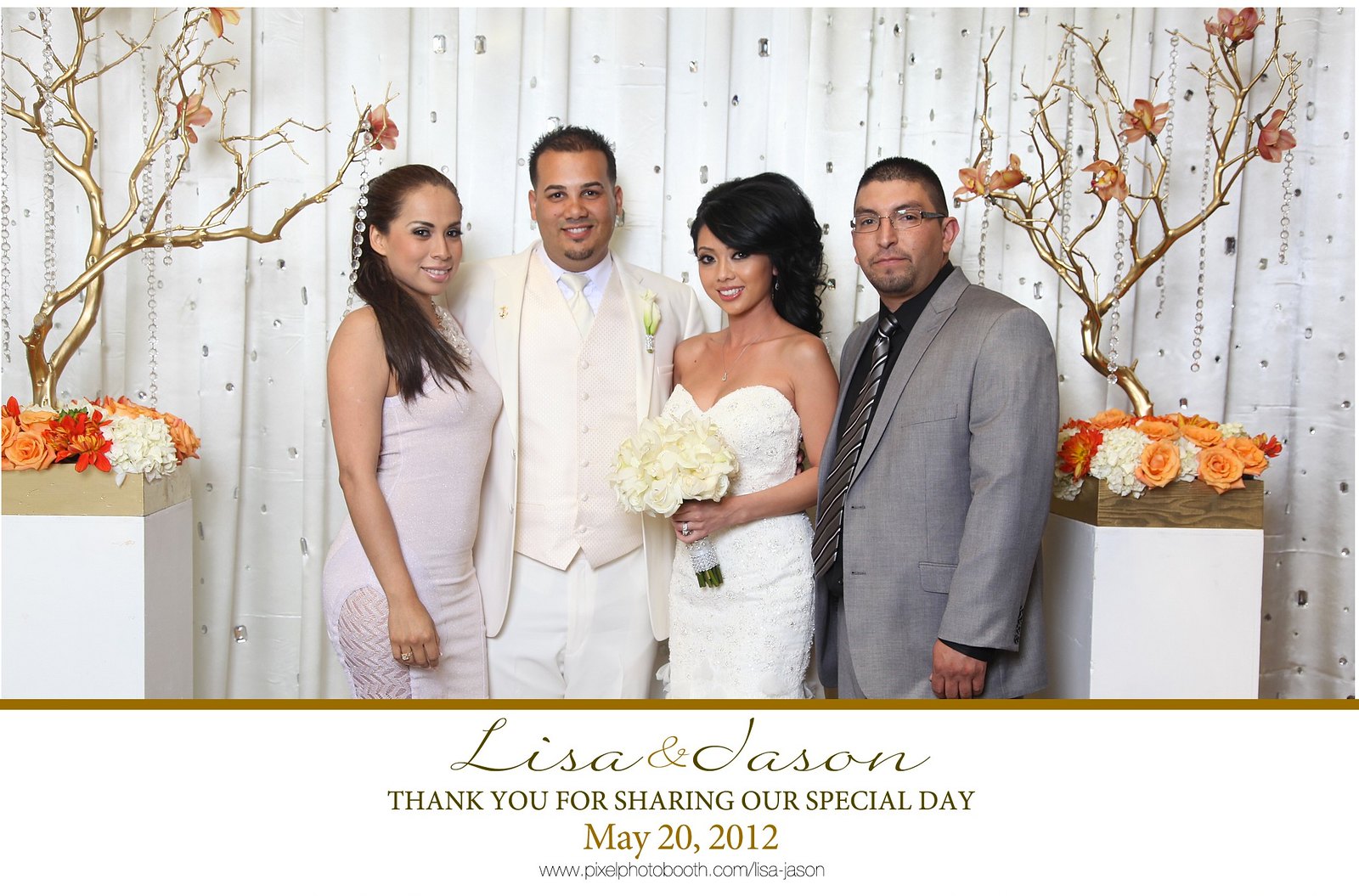This photograph captures a celebratory moment on Lisa and Jason’s wedding day, May 20, 2012, as attested by the white banner at the bottom that reads, “Lisa and Jason thank you for sharing our special day, May 20, 2012, www.pixiephotobooth.com/Lisa-Jason.” The image features four elegantly dressed individuals standing in front of a white curtain adorned with silver teardrop designs framed by ornate flower displays with orange blossoms on golden trees at the edges.

From left to right, the first woman is wearing a tight-fitting sleeveless dress in a very light pinkish cream color. She has brown hair and a tan complexion. Next to her stands a man who appears to be the groom, dressed in a white wedding suit comprising a white vest, formal jacket, collared button-up shirt, tie, and pants. He has short brown hair, tan skin, and a slight goatee with a beard.

The bride, positioned next to the groom, wears a strapless white wedding dress with a sweetheart neckline and holds a bouquet of pale yellow flowers. She has jet-black hair that is elegantly styled up and possesses striking Asian features. The man to her right is wearing a gray suit jacket, a silver black and white tie, and a black collared shirt underneath. He has a lighter complexion, could be Hispanic or white, and is wearing glasses.

Together, these details vividly capture the scene of Lisa and Jason’s wedding, highlighting the stylish attire, the joyful participants, and the celebrative environment.